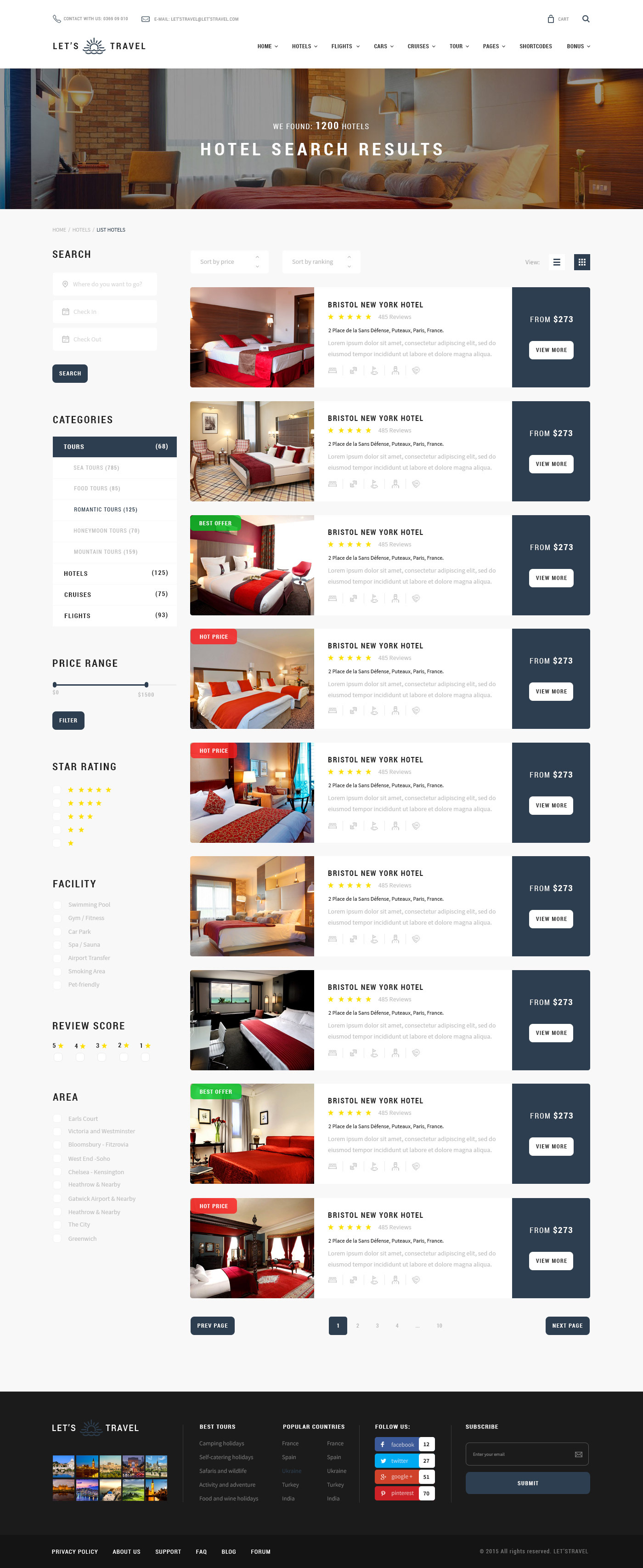The image displays a travel-focused website. In the upper right corner, there is a login button adjacent to a magnifying glass icon, likely for the search function. The top menu bar features a "Home" tab alongside other options such as "Cars" and "Rooms." The header section includes a banner showcasing a hotel room, with the text "Hotel Search Results" prominently displayed in the center.

Below the banner, the page lists nine search results. Each result comprises a room photo, price details, a brief description, and a star rating review. The overall layout is compact and features multiple elements, making the image appear somewhat condensed.